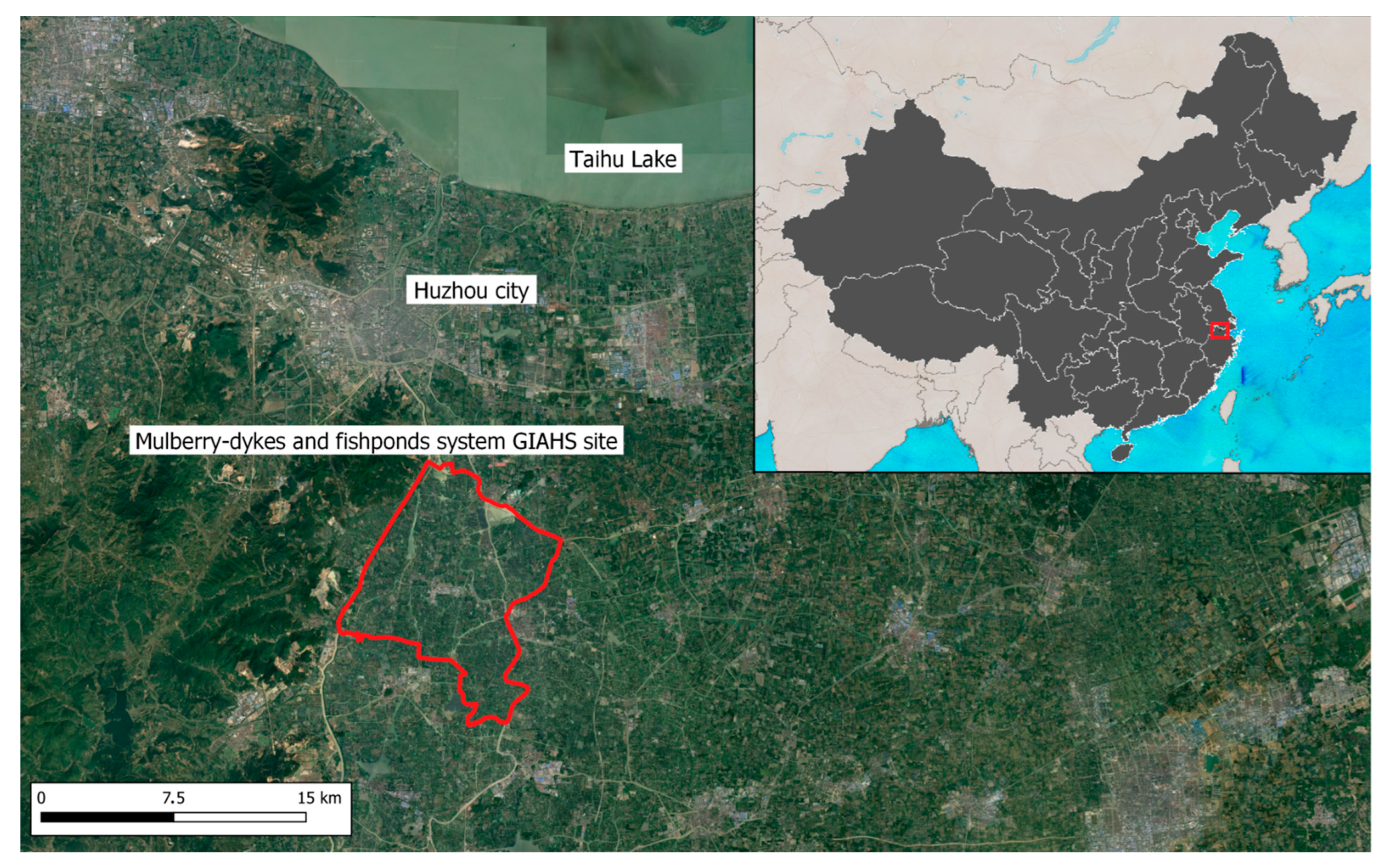The image features a detailed satellite view of a region in southeast China, with Taihu Lake and Huzhou City prominently labeled against a predominantly green backdrop. This satellite image, which occupies approximately 75% of the frame, showcases lush greenery and is highlighted by a red outline marking the "Mulberry Dykes and Fish Pond System, GIAHS site." The top right corner inset provides a broader geographical context, displaying a full map of China with the specified region enclosed in a red square around the lower-right area, along the water. A legend on the left side of the map indicates a scale of 0, 7.5, and 15 kilometers, suggesting the map's zoom level, with black indicating the closest range. Key labels such as "Taihu Lake" and "Huzhou City" appear in black text within white boxes, though "Taihu Lake" is slightly blurred. The combination of satellite imagery and geographic markings provide a comprehensive view of this culturally significant and picturesque area in China.